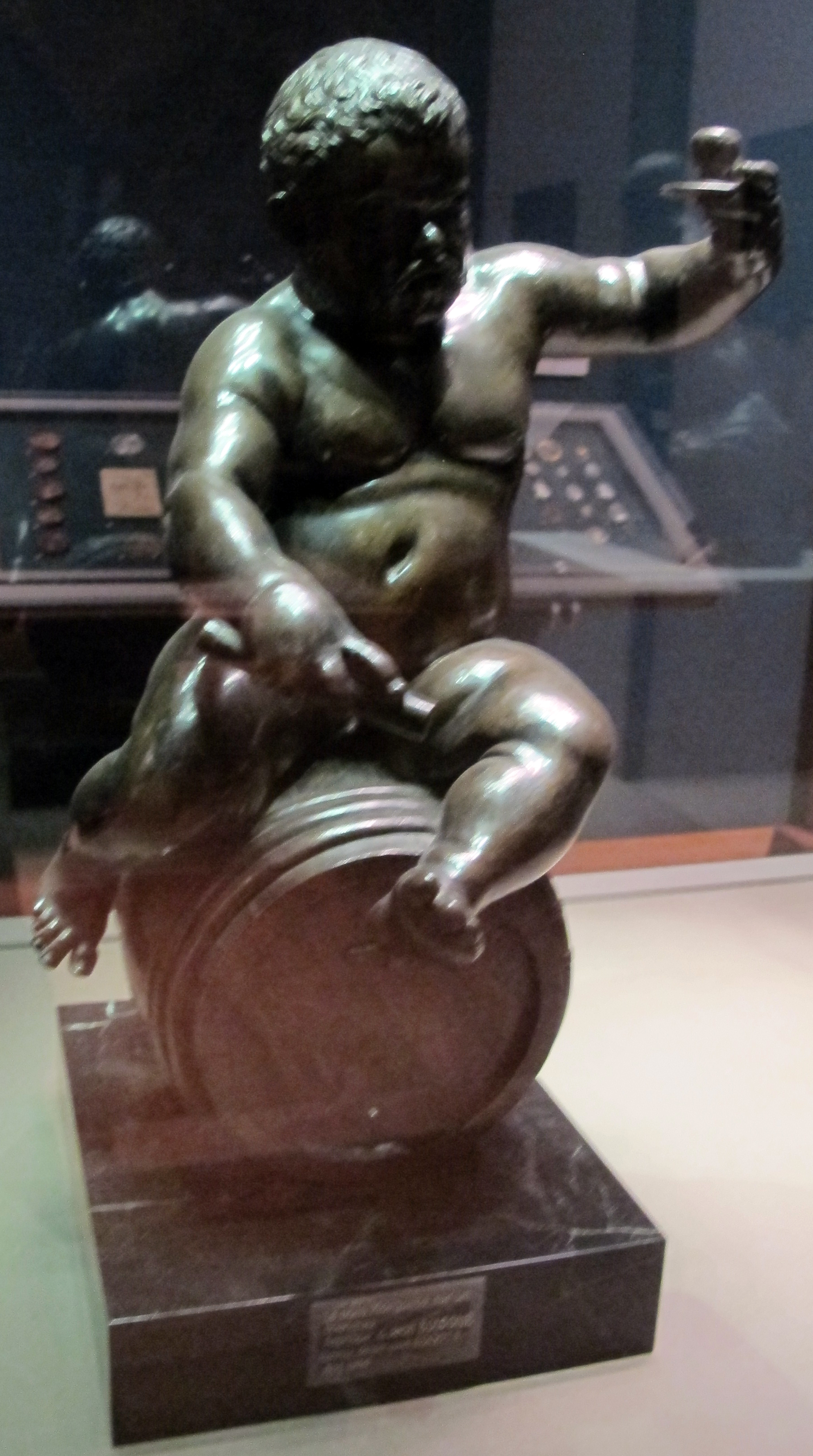The photograph captures a museum display encased in plexiglass, showing a statue situated on a white table with a black marble base. The base features a silver placard, although the text is unreadable. The statue itself is a dark, almost black bronze figure of an overweight, naked man with cropped hair. The man is perched on a sideways-turned barrel, with his left leg draped over the top and right leg extended down the side. His left arm is raised, holding an ambiguous object, possibly a pipe or similar item, while his right hand, appearing to grasp a flute or key, is positioned in front of him. The glare and reflections from the plexiglass reveal additional museum artifacts in the background.